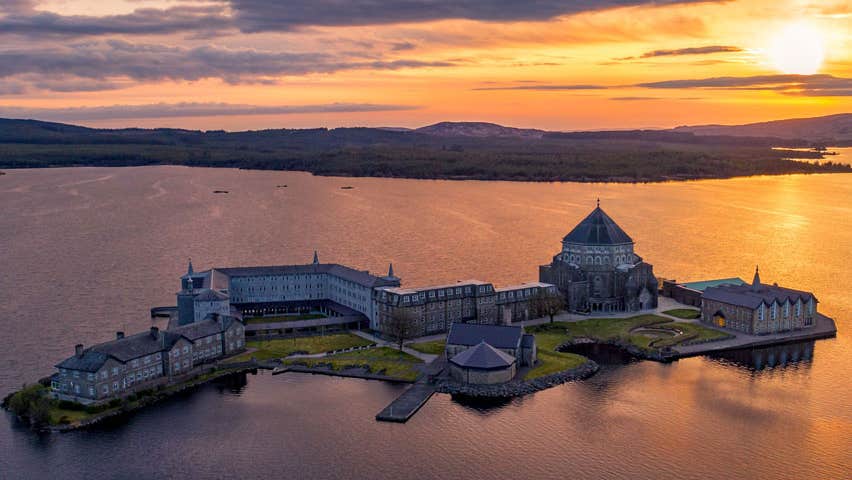This vivid sunset photograph, taken from a bird's eye view, captures a narrow, man-made island in the middle of a large lake or river. The island, less than a mile long and half a mile wide, is densely populated with interconnected, ancient buildings creating a cohesive estate-like complex. 

On the left side, a long, two-story building with a peaked roof and numerous chimneys stretches along the island's length. At the upper edge, a white structure featuring turrets and towers encloses a courtyard. This section merges into a large, round building with a prominent pointed roof, suggesting the presence of a central place of worship, possibly marked by a cross at its pinnacle. 

Adjacent to this, on the right, is a structure characterized by a series of five peaked roofs. A smaller, circular building with an attached pier is noticeable in the foreground, near the shoreline. The foreground buildings are lower, allowing a clear view of the green grass on the shore. 

Behind the island, the serene expanse of water reflects the orange, gold, and purple hues of the setting sun, which is positioned in the upper right corner of the image. The backdrop reveals flat forested land rising into a mountainous horizon, completing this picturesque scene.